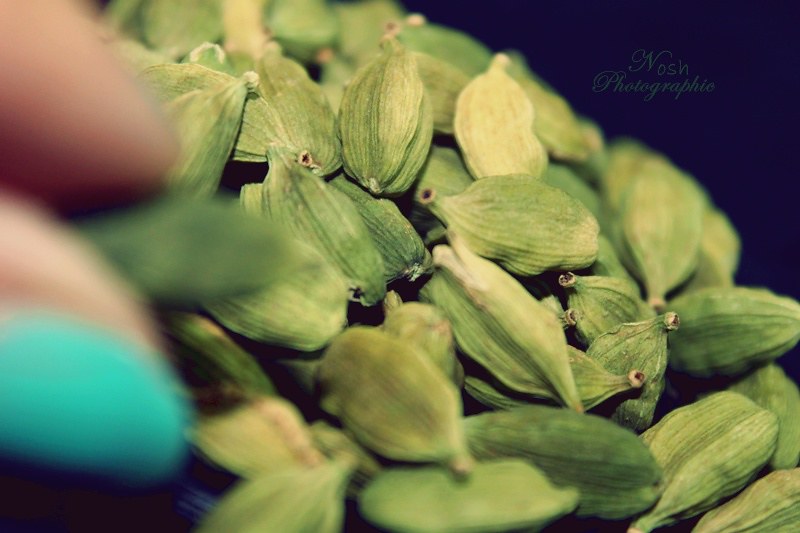This photo captures a close-up of several green, almond-shaped vegetables, likely beans still in their pods, gathered in a central cup-like container. The focal point is the cluster of these vibrant green pods, which have small stem parts still attached. To the left side, there is a blurred image of a hand with blue-painted nails, adding some human interaction to the scene. In the upper right corner, there is a watermark that reads "NOSH Photographic" set against a dark, possibly black, background. The overall color palette includes various shades of green, light blue, tan, and navy blue, suggesting a dramatic contrast. The setting appears to be outdoors, potentially at night, which lends the image a rustic and natural ambiance.